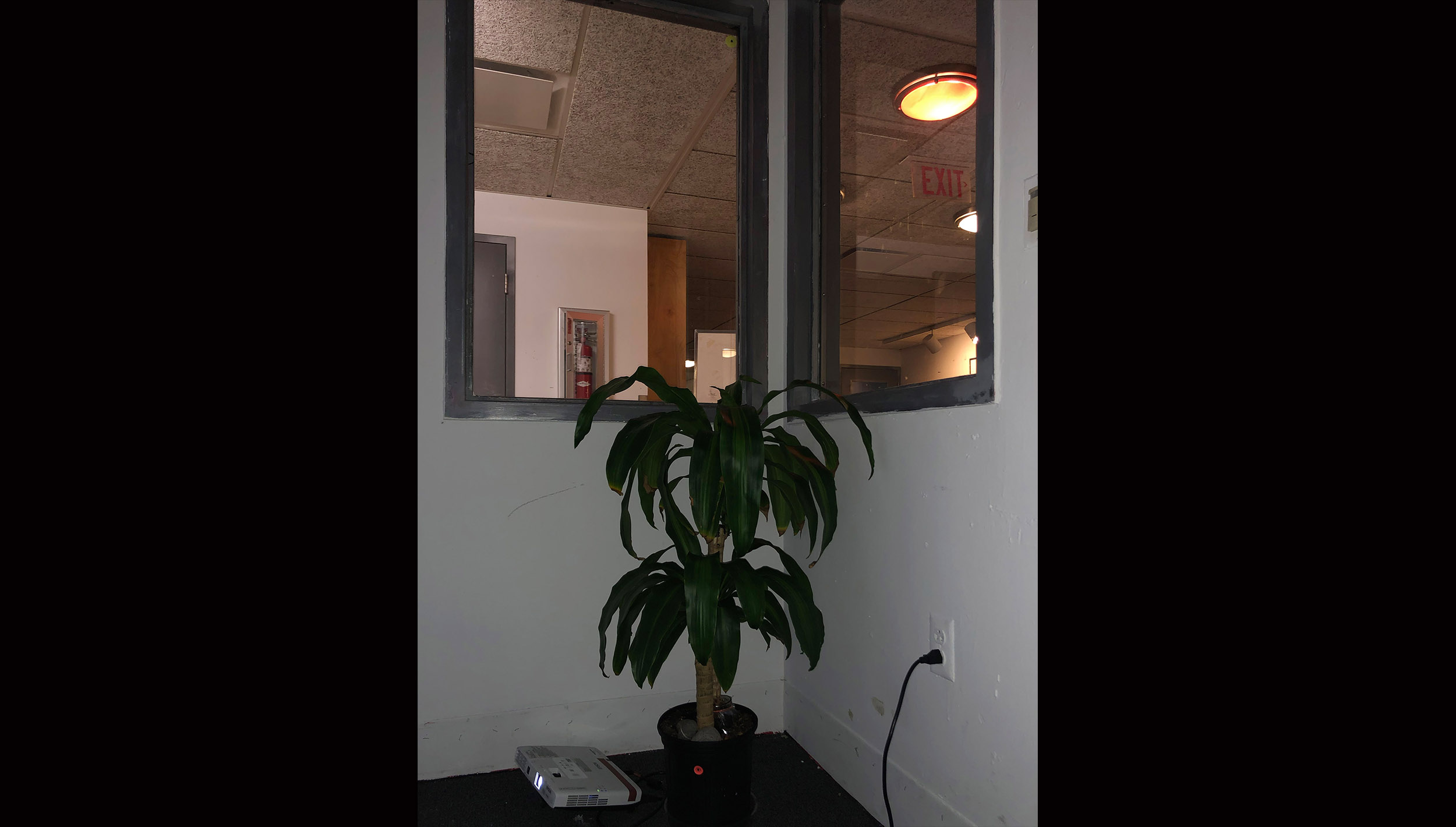This indoor photograph is divided into three distinct sections. Both the leftmost and rightmost thirds of the image present an impenetrable black background, offering no discernible details. The central section, which occupies approximately 40% of the frame, exhibits a more detailed scene. Here, two walls converge at a corner, their surfaces painted in a light beige or whitish hue. The floor below is dark, possibly a deep brown or black, and a portion of it is visible at the bottom center of the photograph.

Adjacent to the corner, there is a rectangular package resting on the floor. Near this package, a potted plant stands, housed in a plain black plastic pot. The plant, resembling an umbrella tree, features a thick trunk and expansive fronds. A black electrical cord extends from the plant, indicating it is somehow connected to the lower wall outlet on the right side.

The ceiling above, composed of brown tiles, includes a ceiling light. The word "EXIT" is noticeable, seemingly reflected or visible through a window. Two windows are apparent, one on each side of the corner junction. To the left of the image, a fire extinguisher is encased behind glass, hinting at the functional aspect of this space. The general ambiance suggests that the scene is set within an office building, complete with hallways and office spaces visible beyond the central plant.